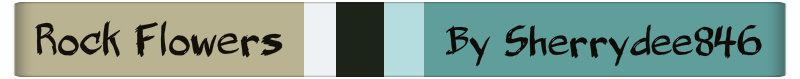The image is a wide, thin banner composed of five distinct vertical sections. On the far left, there's a light brown panel featuring the title "Rock Flowers" in a roughly scrawled black font that resembles crayon or knife carvings. Moving right, a narrow white stripe separates the brown panel from a slightly wider black stripe, followed by a light blue stripe that is wider than the white one but narrower than the black. The far-right section of the rectangle has a teal (or greenish-blue) background with the text "By SherryD846" written in a similar black, crayon-like font. Overall, the banner reads "Rock Flowers By SherryD846" from left to right, with each section contributing to a simple yet colorful design.